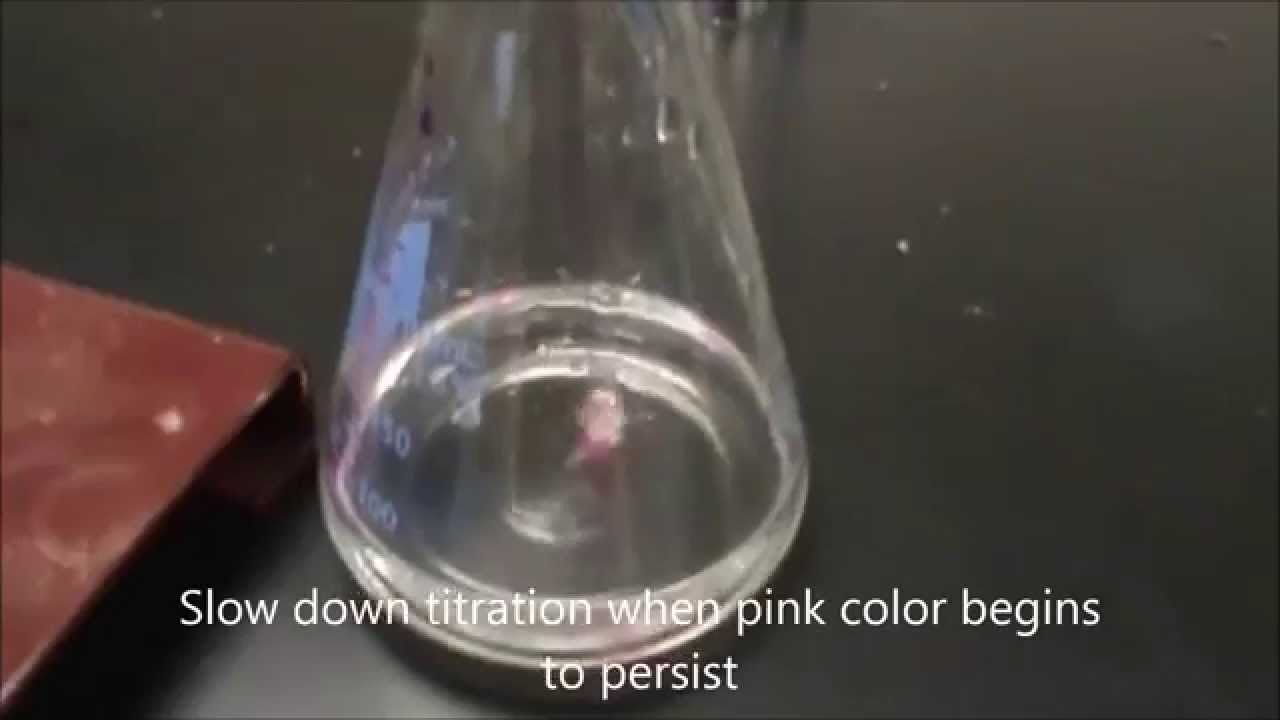In the photograph, a clear scientific beaker takes center stage, prominently displaying measurement markings along its side. The beaker contains a pinkish-hued liquid and rests on a black table or counter that is noticeably speckled with white debris. The beaker is positioned next to a partially visible brown object, possibly a notebook or brick-like material, trailing off the edge of the image. Scattered reflections can be seen, including possible reflections from a computer screen or numerical figures on the left-hand side of the beaker. At the bottom of the image, white font instructions read, "slow down titration when pink color begins to persist," indicating a step in a titration process.